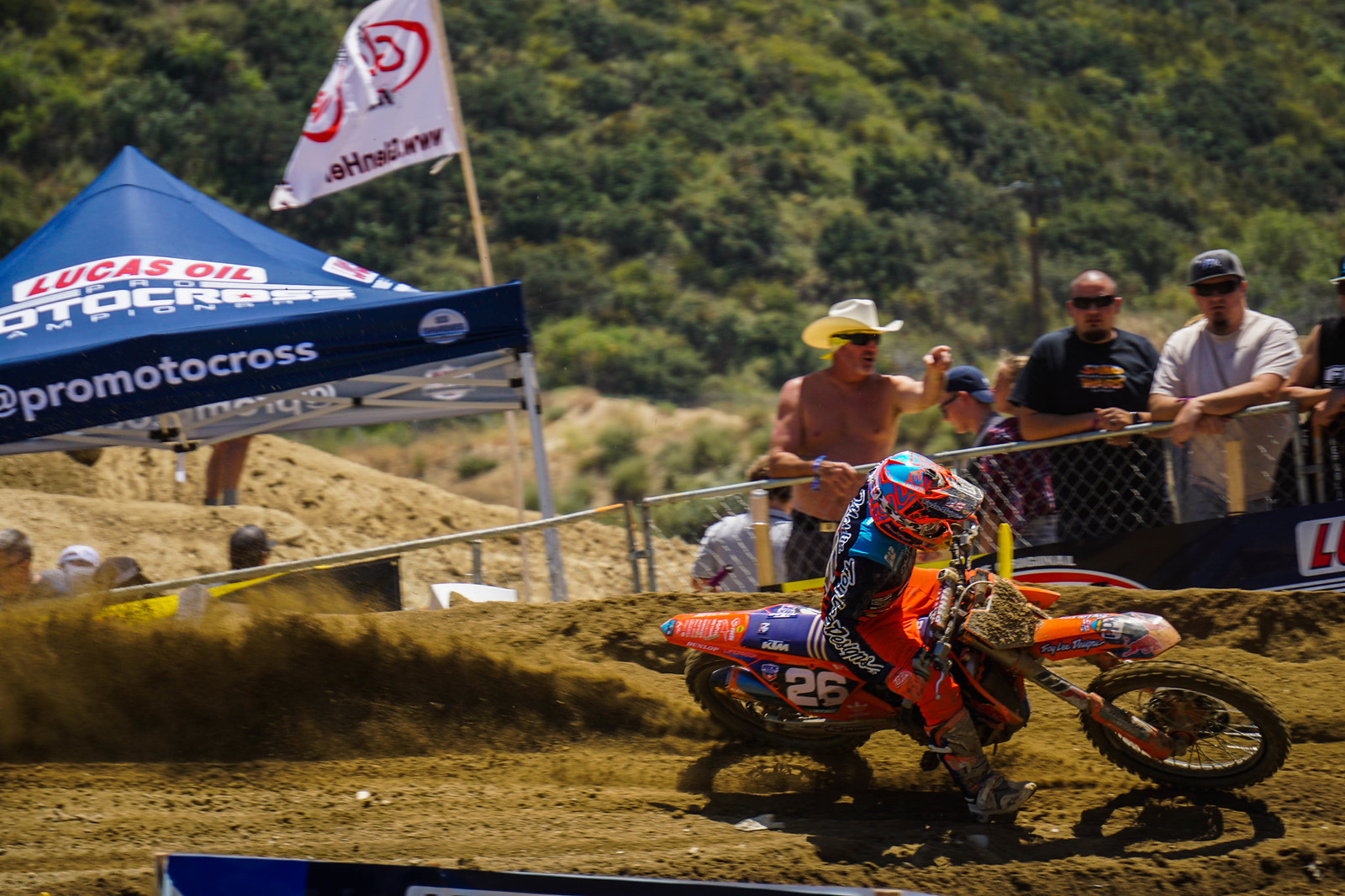In this vibrant, full-color photograph taken during the day at an outdoor dirt bike racing event, a motocross racer is captured mid-race on a winding, muddy track, leaning his orange motorcycle, which bears the number 26, to the right. The rider is clad in orange pants, a long-sleeved blue and black jersey, and a multicolored helmet. Dirt is spinning behind him, emphasizing the intensity and speed of his maneuver. To the left, a blue tent emblazoned with "Lucas Oil Promoto Cross" in red lettering stands prominently, with a white flag waving from its right corner. In the background, tall hills lush with grass and bushes stretch upward, framing the scene. Behind a chain-link fence lining the track, several intent spectators can be seen. They all wear sunglasses, including a shirtless man with a cowboy hat who is pointing at the track, alongside a bald man in a black shirt and another wearing a light-colored shirt.